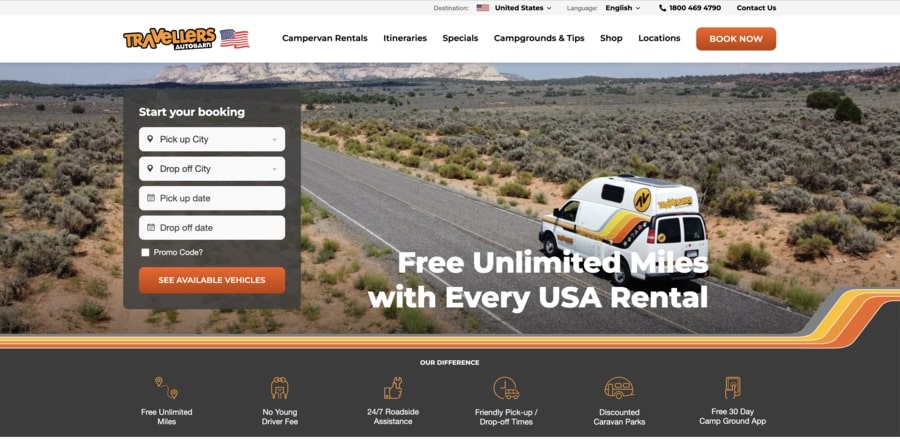This image is a horizontally rectangular screenshot from a website. At the top of the frame, the logo prominently features the word "Travelers" with "Auto" partially visible, hinting at a focus on automotive services. From left to right along the top banner, options include "Camper Van Rentals," "Itineraries," "Specials," "Campgrounds and Tips," "Shop," "Locations," and a "Book Now" button. Beneath this navigation bar, the background image suggests a scenic location likely in the western United States. It depicts a two-lane road stretching into the distance, with a white van traveling towards the upper left of the frame, giving us a rear view of the vehicle. Flanking the road, the landscape consists of sparse short shrubs and dry, dirt-like terrain, characteristic of arid regions. Overlaid on the left side of the image is a window labeled "Start Your Booking," featuring drop-down selections for "Pickup City," "Drop-Off City," "Pickup Date," "Drop-Off Date," a field for a "Promo Code," and a "See Available Vehicles" button.